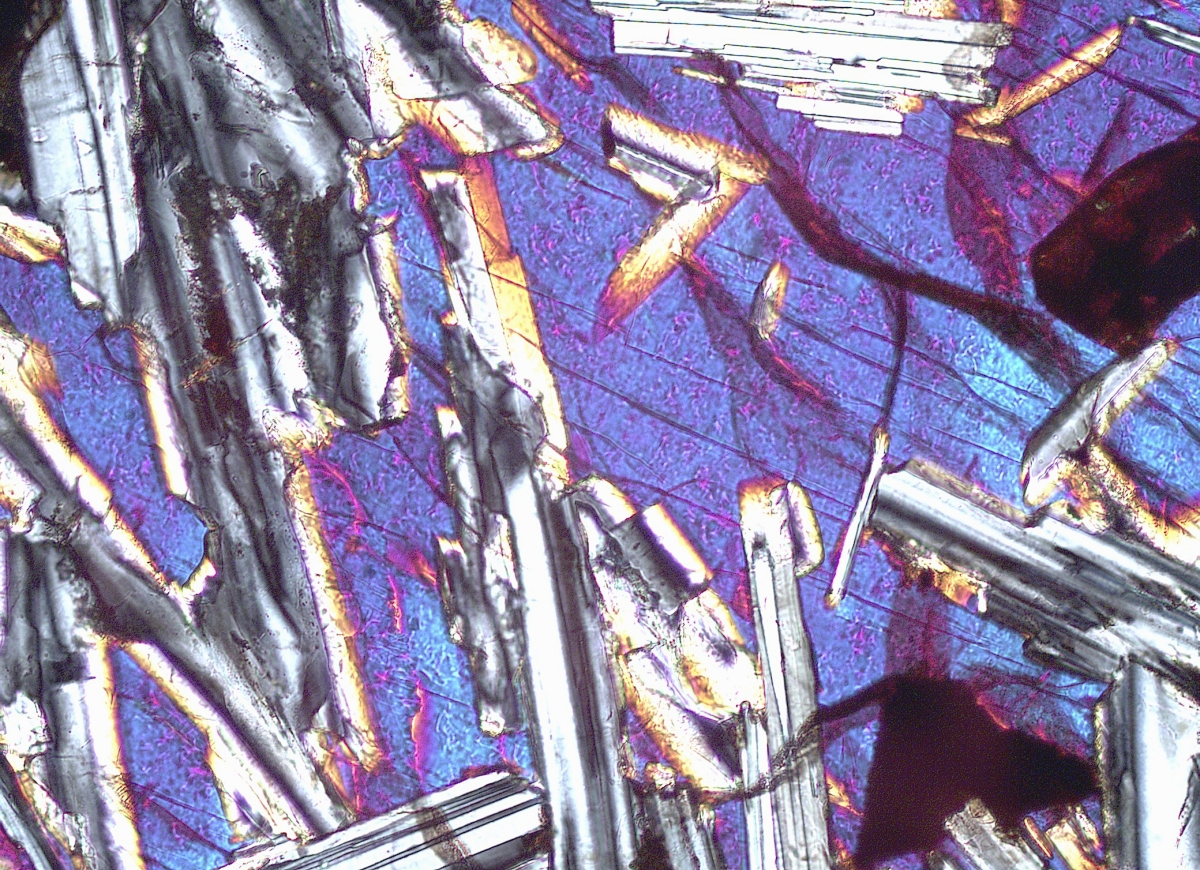This is an image depicting a piece of abstract artwork with a predominant purple-blue background featuring lighter blue areas, predominantly on the right side, intertwined with sporadic red lines. The main focal point is a fragmented metallic structure, primarily gray, with rusty brown hues on some of its components. These shattered pieces vary in size, giving the impression that the fragments are suspended or flying in mid-air. Among the chaotic arrangement, silver rods and elements with orange-yellow borders stand out, adding complexity and depth. The entire composition evokes a sense of disarray and motion, with elements that resemble icicles or ice crystals piercing through the colorful field. Though it is rich in visual detail, the artwork lacks a distinct, identifiable subject, inviting viewers to interpret its meaning through its vibrant, yet abstract, amalgamation of shapes and colors.